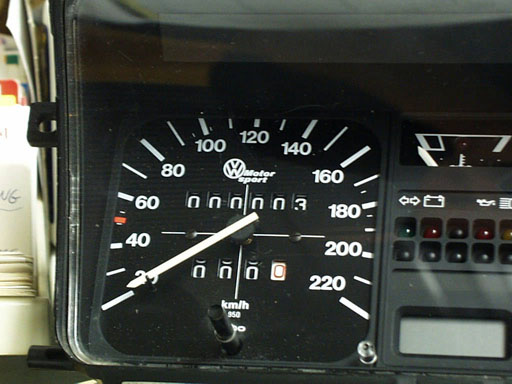The image is a realistic photograph capturing the dashboard of an unidentified vehicle, likely an automotive craft. The dashboard is constructed from entirely black plastic and features a protective glass overlay that prevents direct touch access, ensuring the display is only readable. To the left of the dashboard, white objects and stacked papers are visible in the background, adding context and depth to the scene. 

A small black hoop is affixed to the left side of the dashboard, possibly serving as a handle or attachment point. Centrally positioned on the dashboard is a large black square, dominated by intricate white markings and an attached white needle, indicating its function as a speedometer. The speedometer is calibrated in increments of 20 miles per hour, ranging from 20 to 220 mph in a clockwise pattern. The current reading shows zero miles, suggesting the vehicle is stationary or newly calibrated.

To the right of the speedometer are additional indicators, including a gauge likely displaying fluid levels, as well as dedicated lights for crucial parameters such as battery status and oil level. These features collectively provide comprehensive monitoring of the vehicle’s operational status.